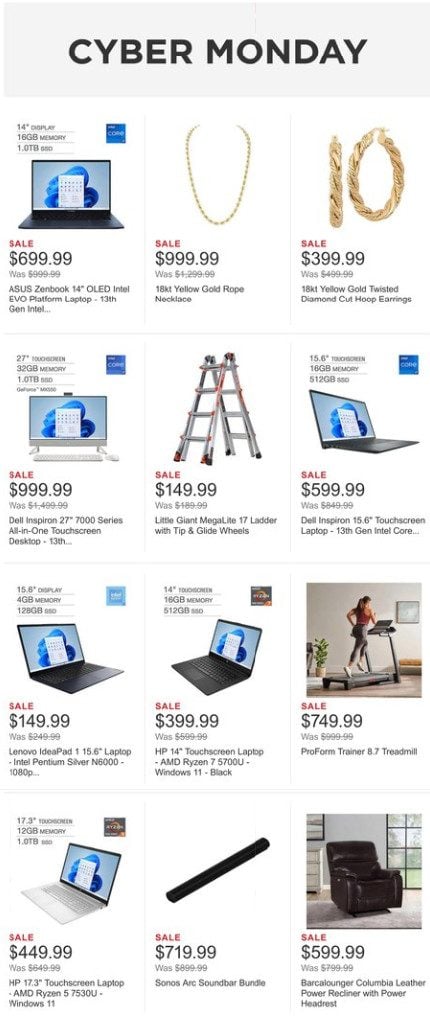The image is a vibrant and enticing Cyber Monday promotional page featuring a variety of discounted items. At the top, a bold banner with "Cyber Monday" in large, black print stands out against a green background. Directly below the banner are eye-catching photos showcasing the available deals.

In the top left corner, there is an image of a computer with the word "SALE" prominently displayed, alongside detailed information about the computer's brand and screen size. Next to it, an image of an 18-karat yellow gold rope necklace highlights a sale price of $999.99. To the right of the necklace, another image advertises 18-karat yellow gold twisted diamond cut hoop earrings on sale for $399.99.

Beneath these featured items, the next row includes three icons: a touch screen desktop, a ladder, and a laptop computer. Further down, another row presents a laptop on sale for $149.99, a touch screen laptop in the center, and a person using a treadmill to the right, highlighting discounted exercise equipment.

The final row showcases three more items: a touch screen laptop on the left, a central image of a sound bar, and a luxurious leather chair on the far right. Each item is clearly depicted, emphasizing the variety and attractiveness of the Cyber Monday deals.